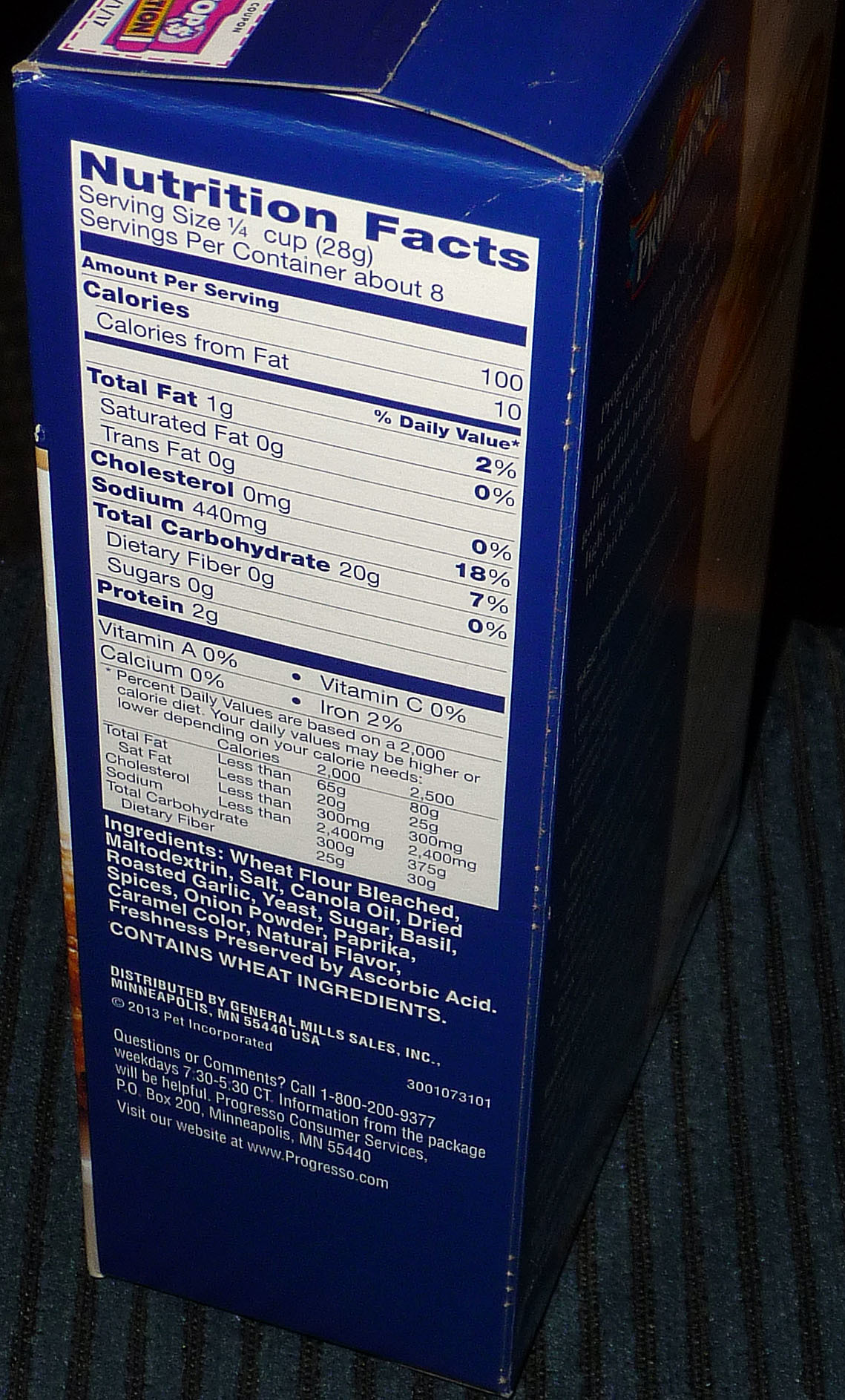This image is a close-up of a blue box displaying a slightly out-of-focus Nutrition Facts label and ingredients list. The label indicates the serving size is ¼ cup (28 grams) with approximately 8 servings per container. The nutritional information includes: 100 calories per serving (10 calories from fat), 1g total fat, 0g saturated and trans fats, along with the amounts for cholesterol, sodium, total carbohydrates, dietary fibers, sugars, protein, vitamin A, vitamin C, calcium, and iron. The ingredients listed are wheat flour, maltodextrin, salt, canola oil, dried garlic, dried spices, onion powder, paprika, yeast, sugar, basil, caramel color, natural flavors, and preservatives like sorbic acid. The label indicates the product is distributed by General Mills, Minneapolis, Minnesota, includes a toll-free number and a website, and possibly belongs to the Progresso brand, suggesting it could be breadcrumbs or a similar product. The white text on the dark blue background makes the nutritional details and ingredients stand out, albeit slightly distorted and hard to read.